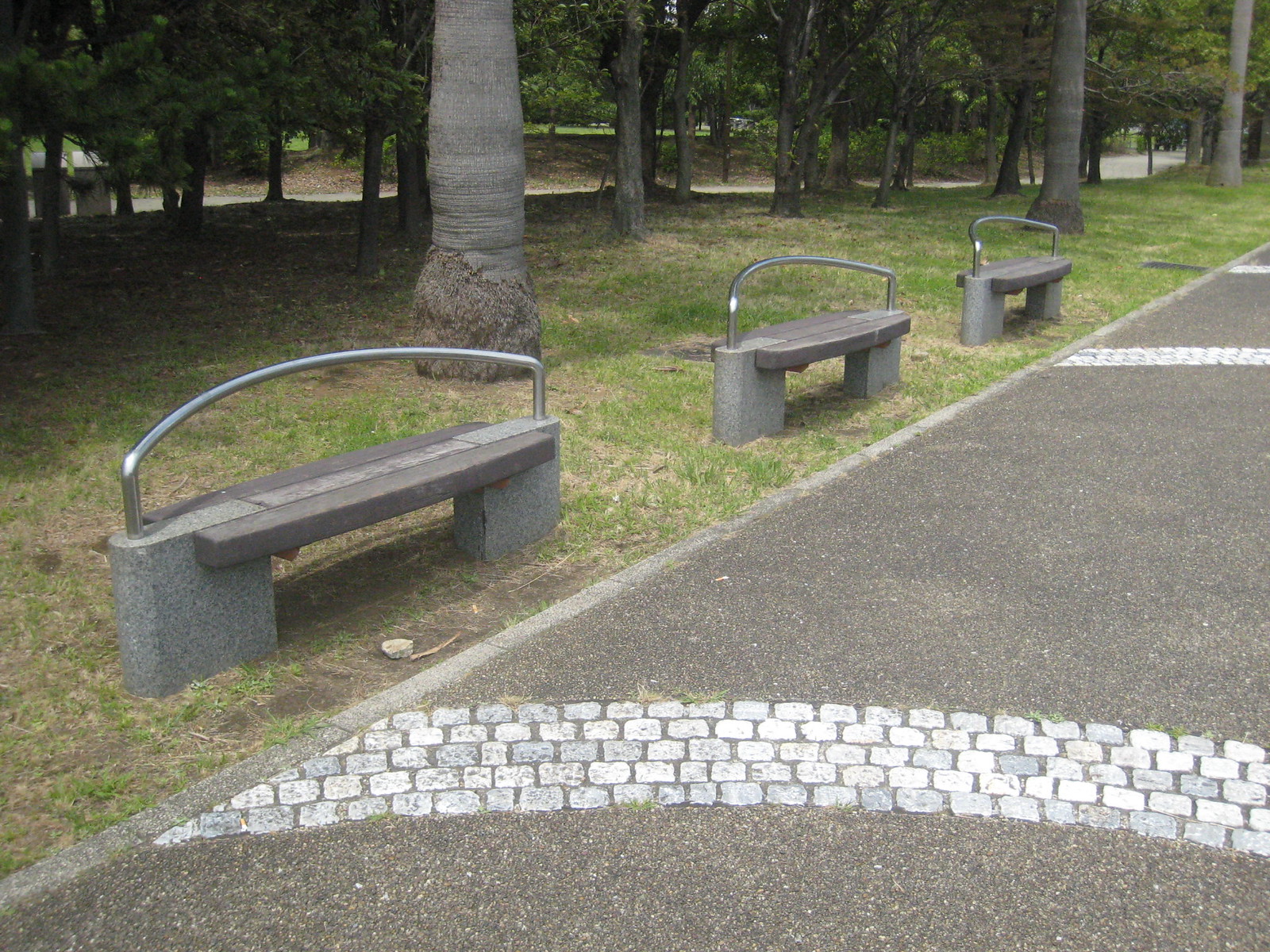This image depicts a tranquil outdoor park designed for exercise and relaxation. On the left-hand side, lush, tall palm trees and other diverse vegetation line a strip of green and brown patchy grass. Central to the image are three distinctive, backless stone benches, possibly made of granite or concrete. Each bench has a stainless steel bar that curves around the back, possibly serving as a backrest or for stretching exercises. These benches are placed in a row along the edge of the grassy area. Adjacent to the benches is a wide, dark grey paved pathway, which appears to be constructed from asphalt with intermittent streaks of cobblestones. This path, currently devoid of pedestrians, curves and follows around the back of the trees, creating a scenic route for walking or running. The park extends further into the background, where a gravel path and more green space can be observed. The overall setting suggests a serene, overcast day, contributing to a calm ambiance.